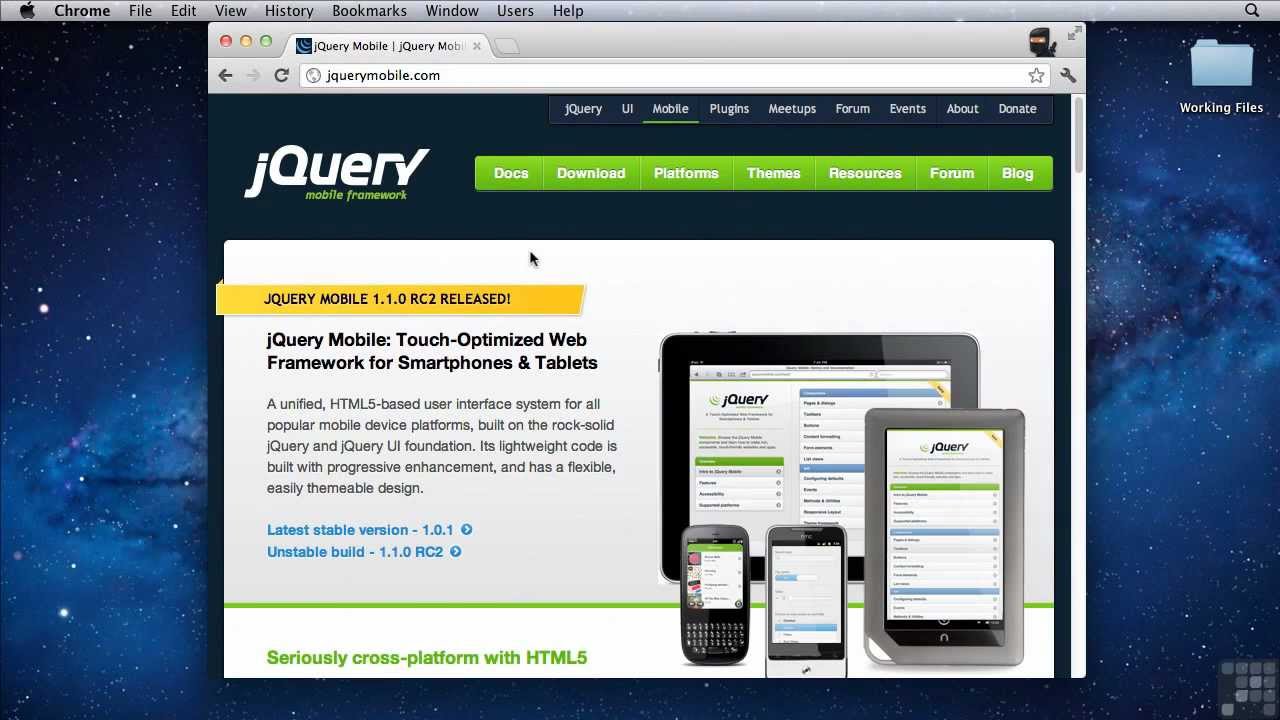In the background of the image, a serene night sky is depicted with a rich gradient from dark navy blue to black in the upper left corner. This celestial canvas is dotted with bright white stars, adding a sense of depth and tranquility. 

Foreground elements are framed within a gray navigation bar, showcasing various options such as Chrome, File, Edit, View, History, Bookmarks, Window, and Help. Beneath this is a search bar containing the uppercase term "QUERY." 

To the right, rendered in a long green rectangle, are labeled options including Docs, Download, Platforms, Resources, Forum, and Blog. Centrally positioned within this section is the word "Theme," indicating a focal area for thematic elements.

Located in the upper right corner, a small blue folder icon juxtaposes against the starry sky, labeled "Working Files" beneath it.

Highlighted in a long yellow rectangle is the announcement: "jQuery Mobile 1.10 RC1 released." Additional text elaborates, describing jQuery Mobile as a touch-optimized web framework for smartphones and tablets, emphasizing its role as a unified HTML-based user interface system catering to all popular mobile device platforms.

The image further features visual examples of this program displayed on an iPad and a cell phone, reinforcing its compatibility and user-friendly design for mobile devices.